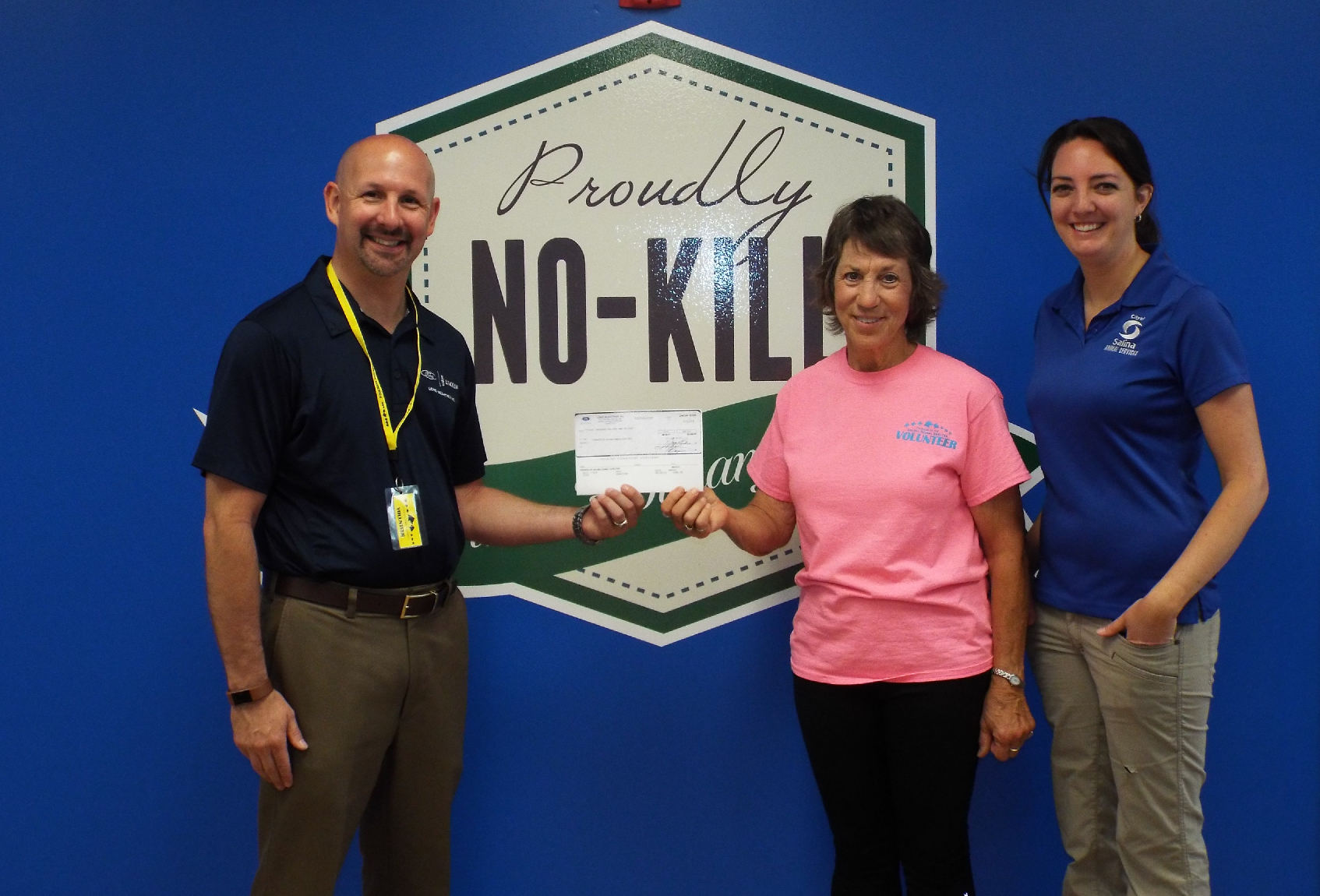In this vibrant photograph, three smiling individuals stand in front of a blue banner proudly displaying a "Proudly No-Kill" logo, signifying support for a no-kill animal shelter. On the left, a bald man with a yellow lanyard, dressed in a black shirt with a brown belt and khaki pants, extends a white check towards an elderly woman. She stands on the right, joyfully accepting the donation, dressed in a pink shirt and black pants. To her immediate left, a younger woman with black hair, wearing a blue polo shirt with a logo and khaki pants, stands with her hands in her pockets. The image captures a moment of support and camaraderie for the animal shelter, underscored by the shared smiles and the generous act of giving.